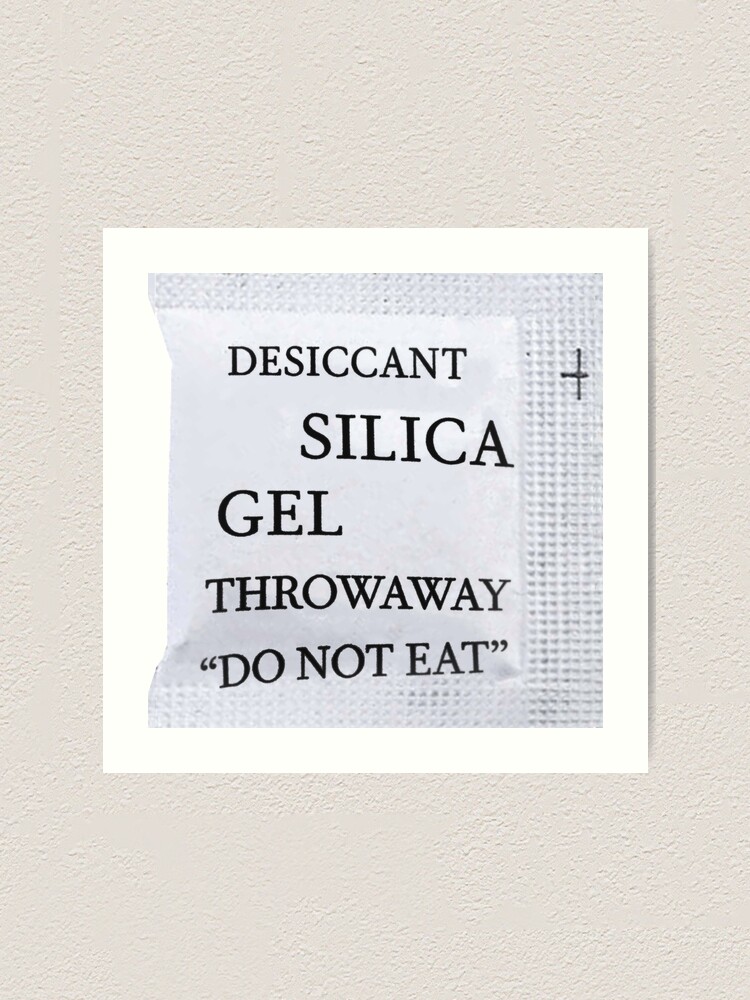This detailed photograph captures a framed artwork, prominently featuring a silica gel packet against a white background. The artwork, which appears square-shaped, is centered on a cream or off-white textured wall. The silica gel packet, shown in dark gray, is crimp-sealed and bears the text in black letters: "DESICCANT", "SILICA", "GEL", "THROW AWAY", and "DO NOT EAT" in quotation marks. The packet is set on a white card that serves as the background for the piece, surrounded by a white border that further emphasizes the stark contrast between the packet and the background. The overall image has a monochromatic appeal, highlighted by the textured wall and the detailed presentation of the silica gel packet. The landscape orientation of the photograph helps to capture the entirety of the framed artwork and its placement within the room.